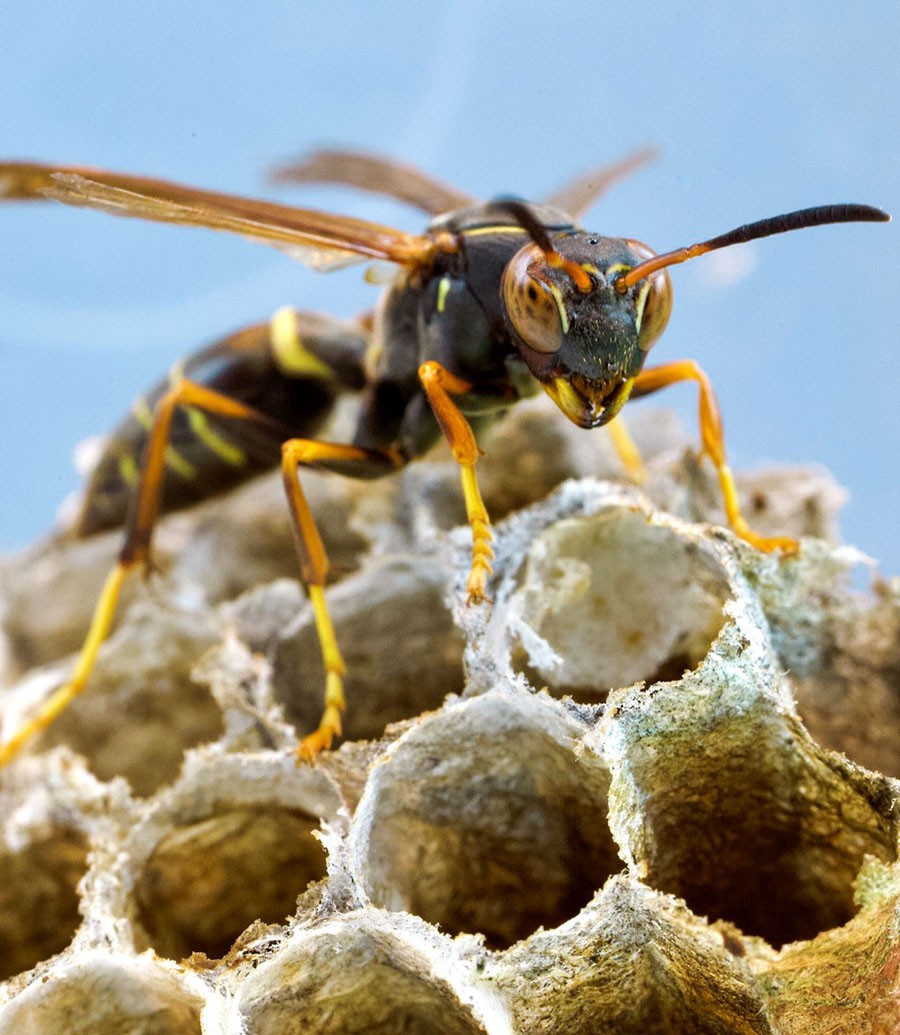In this highly detailed macro photograph, a wasp, often mistaken for a hornet or yellowjacket, is featured in extreme close-up, showcasing its intricate details. Perched atop a dry, circular honeycomb-like nest, the wasp displays its striking coloration. The wasp's body is predominantly brown to almost black with vivid yellow stripes adorning its back. It has five visible orange legs and two long antennas that are orange at the base and transition to black. The head of the wasp, featuring large, brown compound eyes, is turned towards the camera, seemingly making eye contact. The wings, also brown, are spread slightly, giving a glimpse of its readiness to take flight. The background of the image is a clear blue sky, enhancing the natural beauty of this detailed insect study. The image’s composition and clarity bring an intimate view of the wasp and its nest, emphasizing the natural world's complexity and beauty.